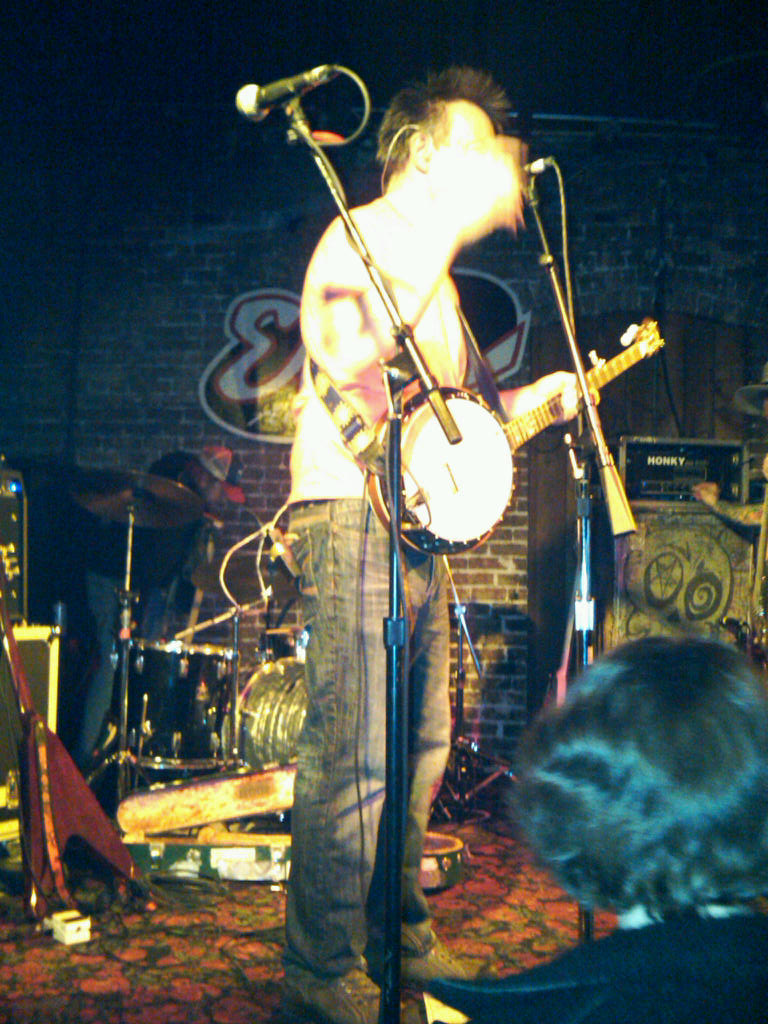In the image, a musician is performing on a dimly lit stage, likely in an underground club or bar with a brick wall backdrop adorned with graffiti partially obscured by the performer. He holds a five-string banjo with a white center and black outline, the neck of a bamboo-brown hue. Clad in a white short-sleeve shirt and light blue jeans, along with brown boots or sneakers, he also has black, spiky hair styled into a frohawk. A microphone in front of him captures what appears to be a solo performance, as his raised hand with a shaker obscures his face. The stage is surrounded by various musical instruments, including a drum set, several guitar and banjo cases, a guitar amplifier, and possibly a balalaika or mandolin. A single audience member is visible in the bottom right corner, a woman with fluffy, curly black hair wearing a black coat with a long collar. The floor is carpeted in dark hues with a red floral pattern, contributing to the intimate ambiance of the setting.